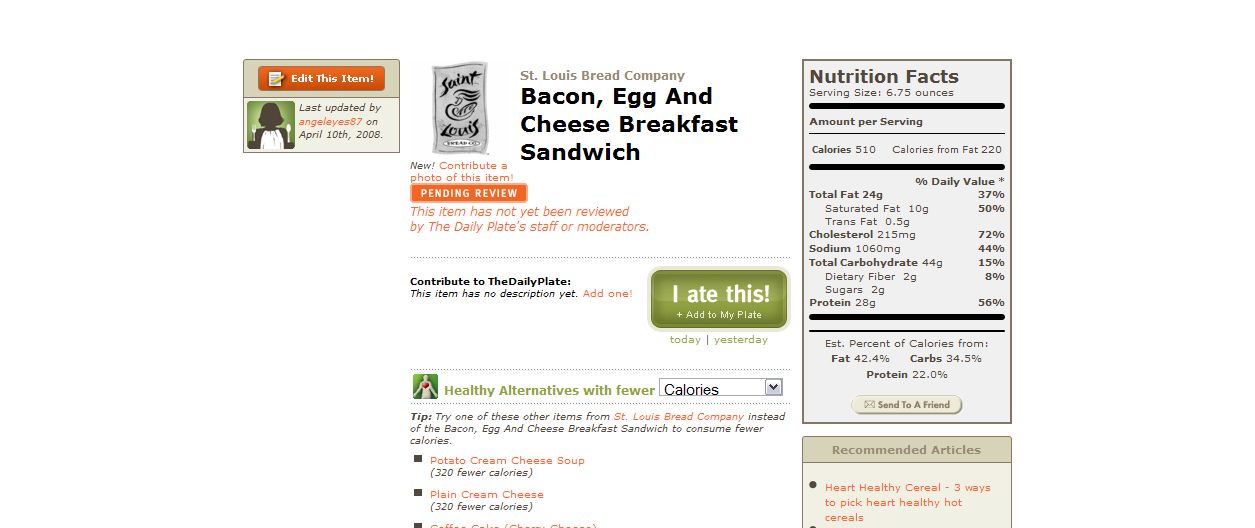The image is a detailed screenshot from a food tracking app used to monitor daily caloric and nutritional intake. The highlighted item being analyzed is the Bacon, Egg, and Cheese Breakfast Sandwich from the St. Louis Bread Company. In the center of the screen, a prominent green button labeled "I Ate This – Add to My Plate" allows users to log their consumption of this sandwich. Below the food item, there is a dropdown menu offering options to find healthier alternatives with fewer calories or adjusted nutritional values. The right side of the screen features a section dedicated to the sandwich's nutrition facts, providing an in-depth breakdown of its caloric and nutrient content. Additionally, there is a user-friendly button that enables sharing this information with a friend.